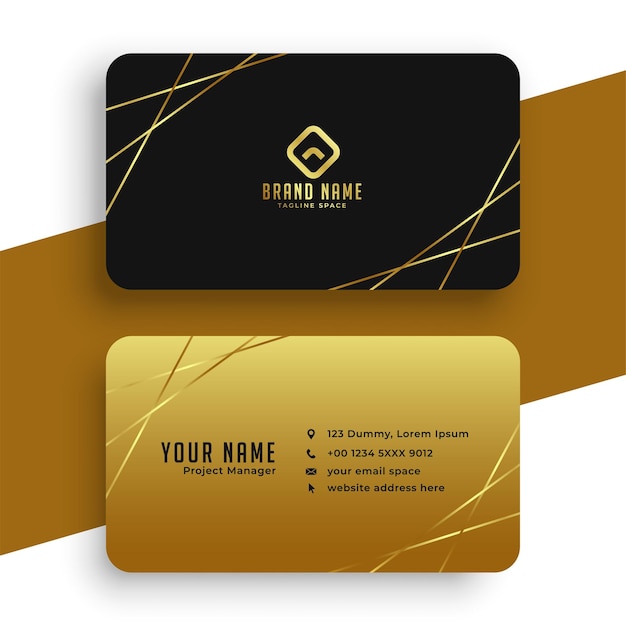The image displays a mock-up of two rectangular business cards with rounded edges, over a gold parallelogram background. The upper card is black, featuring three gold lines crisscrossing the top left and bottom right corners. At the center of this card, a square set on point with a small curve inside houses the text "brand name" and "tagline space" below it. The lower card has a gradient golden tan color, lighter at the top and darker at the bottom, and similarly decorated with crisscrossing gold lines on the corners. The left side of the lower card reads "your name" followed by "project manager." The right side includes icons next to placeholders: a map pin next to "123 dummy Lorem Ipsum," a phone icon next to a dummy phone number, an email icon followed by "your email space," and an arrow cursor icon with "website address here." The backdrop of these cards is a white background intersected by a bronze-colored stripe, enhancing the overall design.